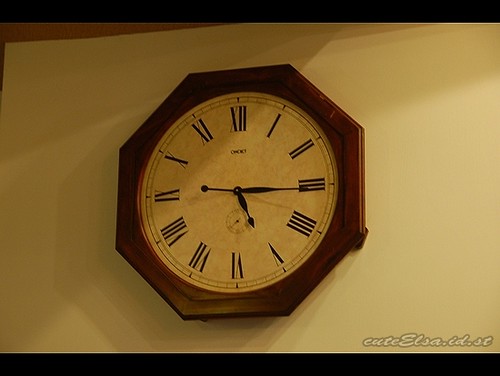This photograph features a stylish wall clock mounted against a pristine white wall. The clock's frame is crafted from hexagon-shaped, rich brown wood, lending it a touch of rustic charm. The clock face is white, punctuated by a subtle circular border that adds an understated elegance. Black metal hands mark the time; both the minute and second hands point to 3, while the hour hand rests on 5. The timepiece features classic Roman numerals, enhancing its vintage appeal. In the bottom right corner of the clock face, a graceful signature in cursive reads "CuteElsa.ld.sc," adding a personalized touch to the design.